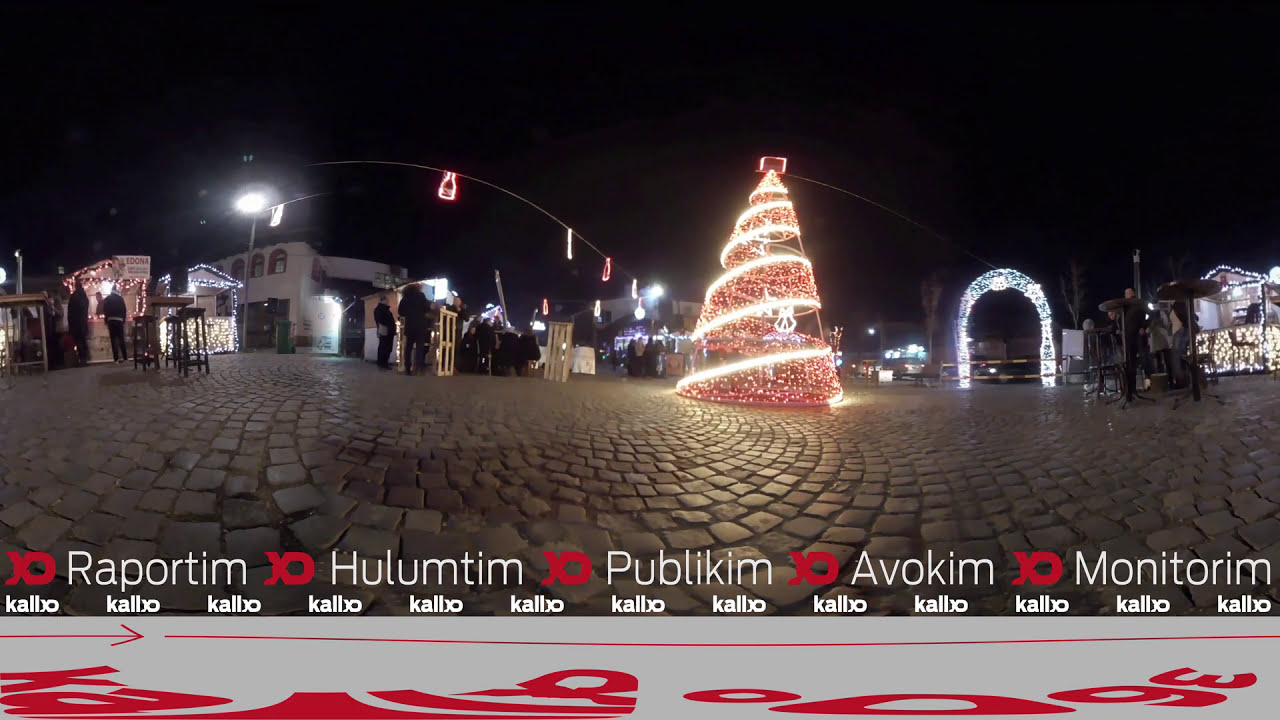This panoramic image captures an enchanting Christmas market set in a cobblestone courtyard at night. Dominating the center is a large, vividly lit Christmas tree adorned with red, white, and yellow spiral lights. Flanking the scene are numerous festively decorated stalls and small buildings, suggesting a range of vendors. A prominent lit arch, illuminated with blue lights, serves as a picturesque entryway to the festive square. Scattered throughout are additional Christmas lights and decorations strung from poles. Clusters of people, tables, and chairs suggest a lively and bustling atmosphere. Text overlays in white reading "rapportim, haleptim, publicim, avokim, monitorim" and a repeating "K-A-L-L-X-O" pattern below add an enigmatic layer to the scene. The bottom gray banner features upside-down red "360 degrees" text and a red line with an arrow, hinting at the panoramic nature of the photograph or a live video feed. The overall ambiance captures the festive joy and communal spirit of a town square adorned for the Christmas season.